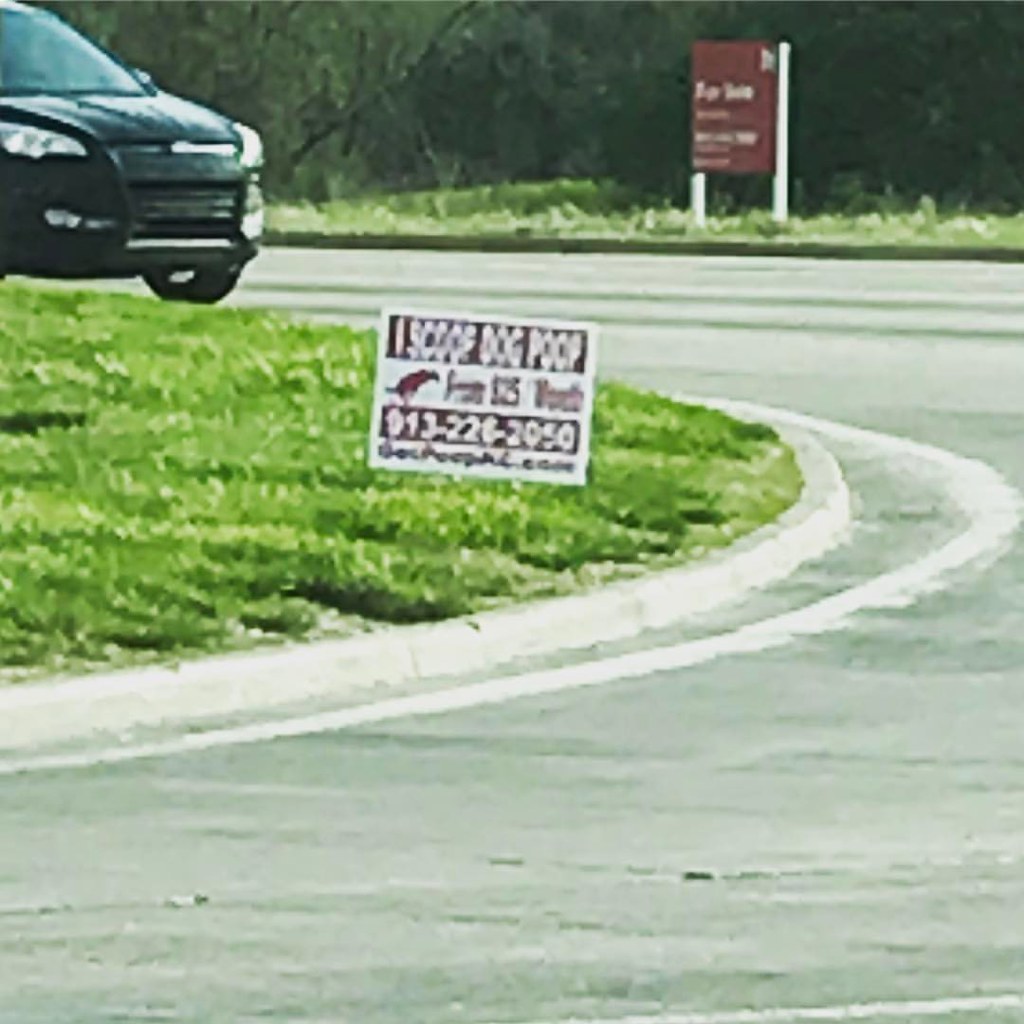This outdoor color photograph captures a black car driving down a light gray road that makes a sharp curve to the left. Flanking the road on either side is a mix of light and dark green grass that is slightly overgrown. In the middle of the image, there's a small berm lined with a concrete edge and marked by a white line around its perimeter. Stationed on the berm, among dark green leaves and foliage, stands a small red sign featuring the white text: "I scoop dog poop." Below this headline, the sign details a service priced "from $25," accompanied by a silhouette of a dog and the contact number "913-226-2050" against a red rectangle. In the background, another red sign with white text is partially visible but unreadable. The trees and plants behind the road contribute to a verdant, natural setting.